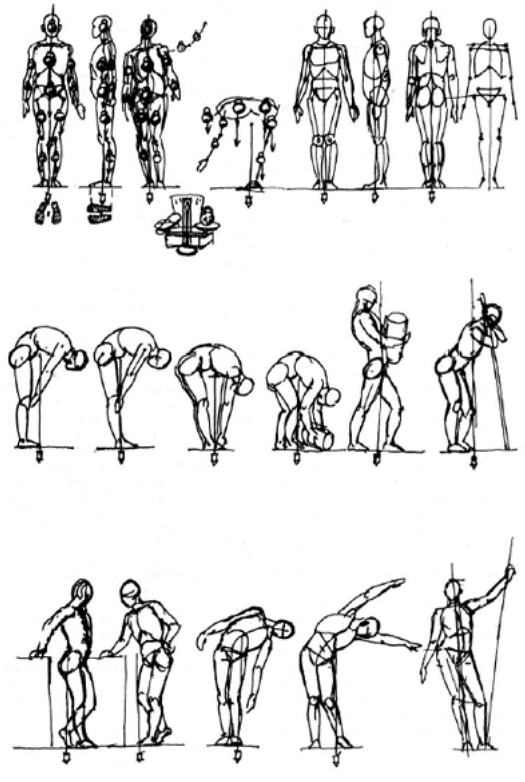The image is a detailed instructional drawing of the human anatomy, intended to guide artists in depicting human figures. It features three rows of black-and-white hand-drawn figures on a white background. 

In the first row, there are five figures demonstrating various poses: front view, side view, back view, and bending over. The figures are gender-neutral and feature circles highlighting significant anatomical points. 

The second row consists of six sequential images illustrating the process of bending over to pick up an object. The sequence begins with slight bending, progresses to picking up a barrel, and ends with the figure standing straight, leaning against a pole.

The third row showcases five more figures in diverse postures: one leaning back against a surface, another leaning on an elbow, another bending sideways to the right, one stretching arms to the right, and the final figure stretching an arm upward. None of the figures have hair, faces, or clothing, reinforcing the instructional focus on body mechanics and movement.